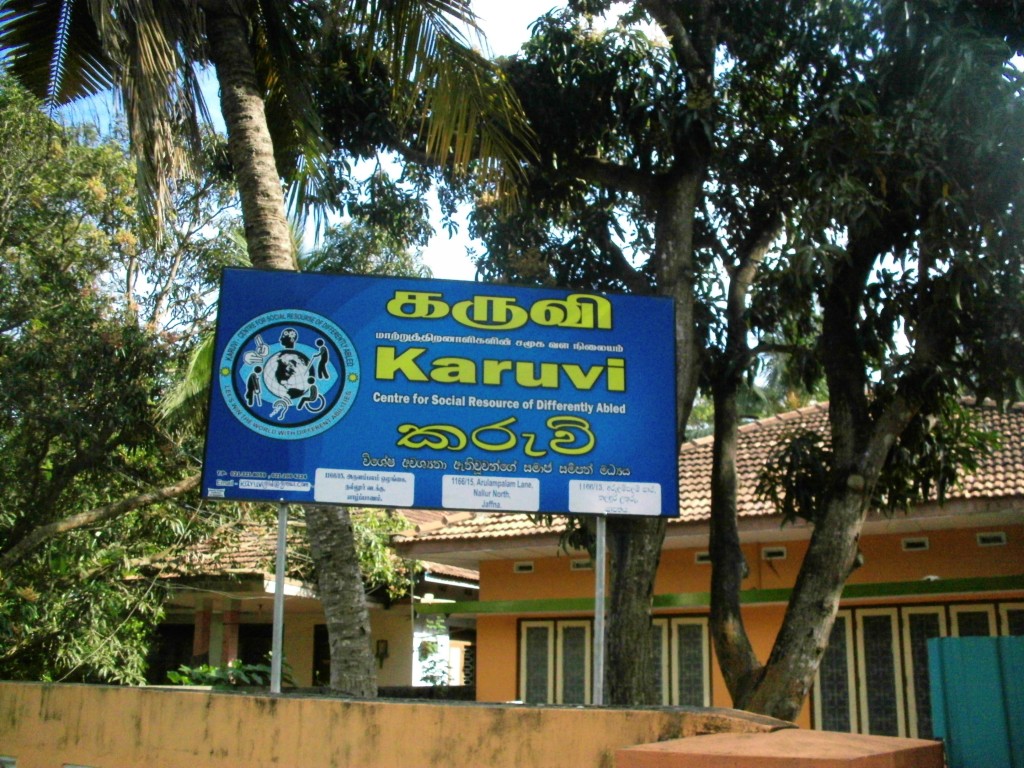The image depicts an exterior scene in what appears to be a possible South Asian or African setting, featuring a prominent sign that reads "Karoovi. Center for Social Resources of Differently Abled," indicating it is a facility for disabled services. The scene is set outside in a residential-looking area with several buildings, some of which are yellow with closed window shades and vent tops. The sign is large and positioned centrally, secured on a cement slab and surrounded by various trees, including tall trees with brown trunks and palm trees. The background shows a blue sky with some clouds visible through the trees. The sign itself is blue with yellow and white text, and it contains a logo featuring people around a globe, possibly forming an eye shape. The colors in the image include shades of white, blue, green, brown, yellow, orange, and light blue. Additionally, there is a green strip on one of the buildings and a light blue object standing in the bottom right corner of the image.